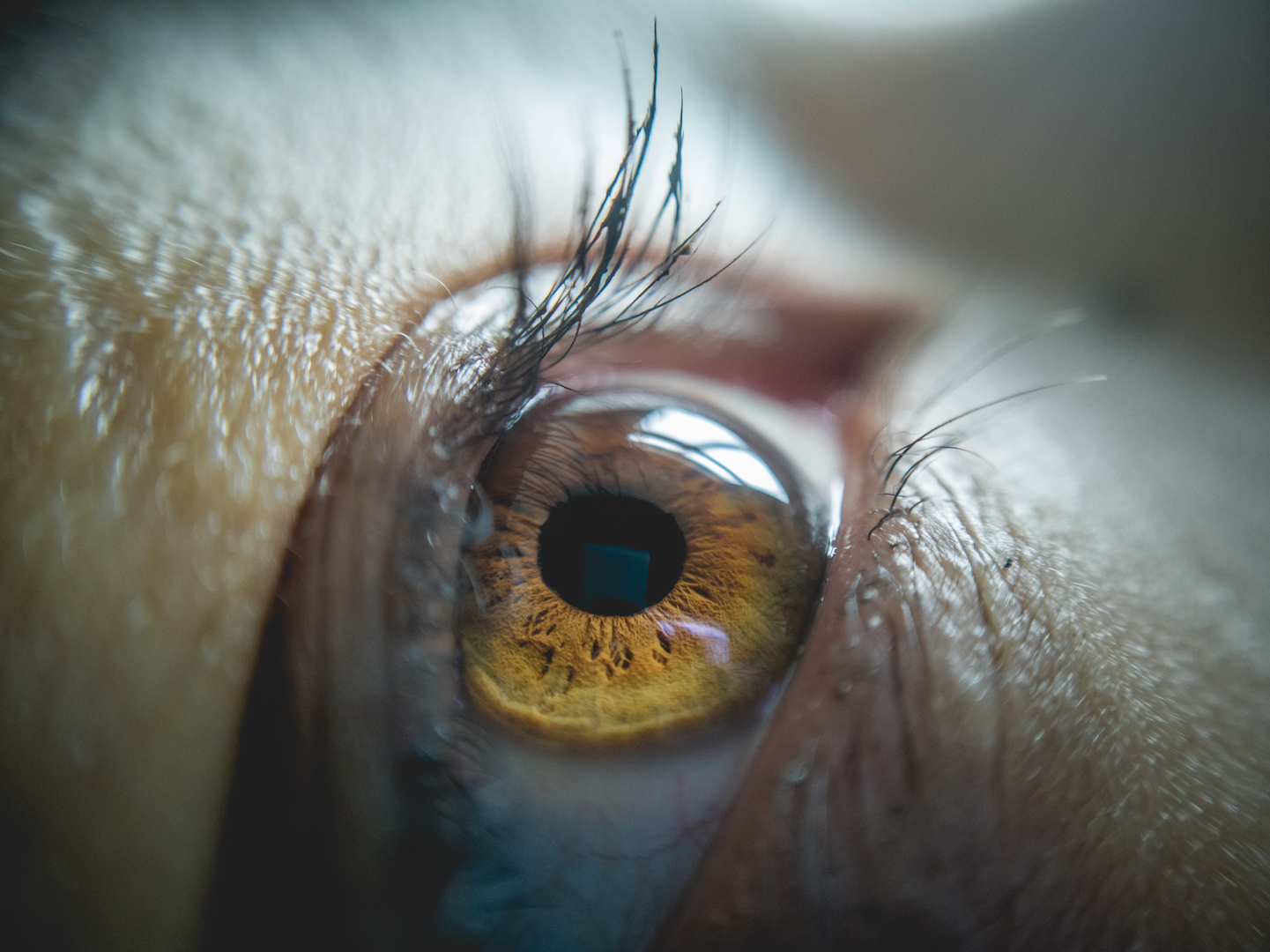This detailed photo captures a close-up of a human eye, specifically what appears to be a female's right eye. The iris is a striking hazel, encircling a black pupil. Her eyelashes are accentuated with mascara, and a natural light source is reflected from a window, creating a soft glow across her eye. The skin around the eye is visible, displaying fine details and subtle textures. Red blood vessels are noticeable in the white part of the eye, particularly near the bottom. The photo, devoid of text, showcases the eye's sharp definition and the natural lighting that highlights its intricate beauty.